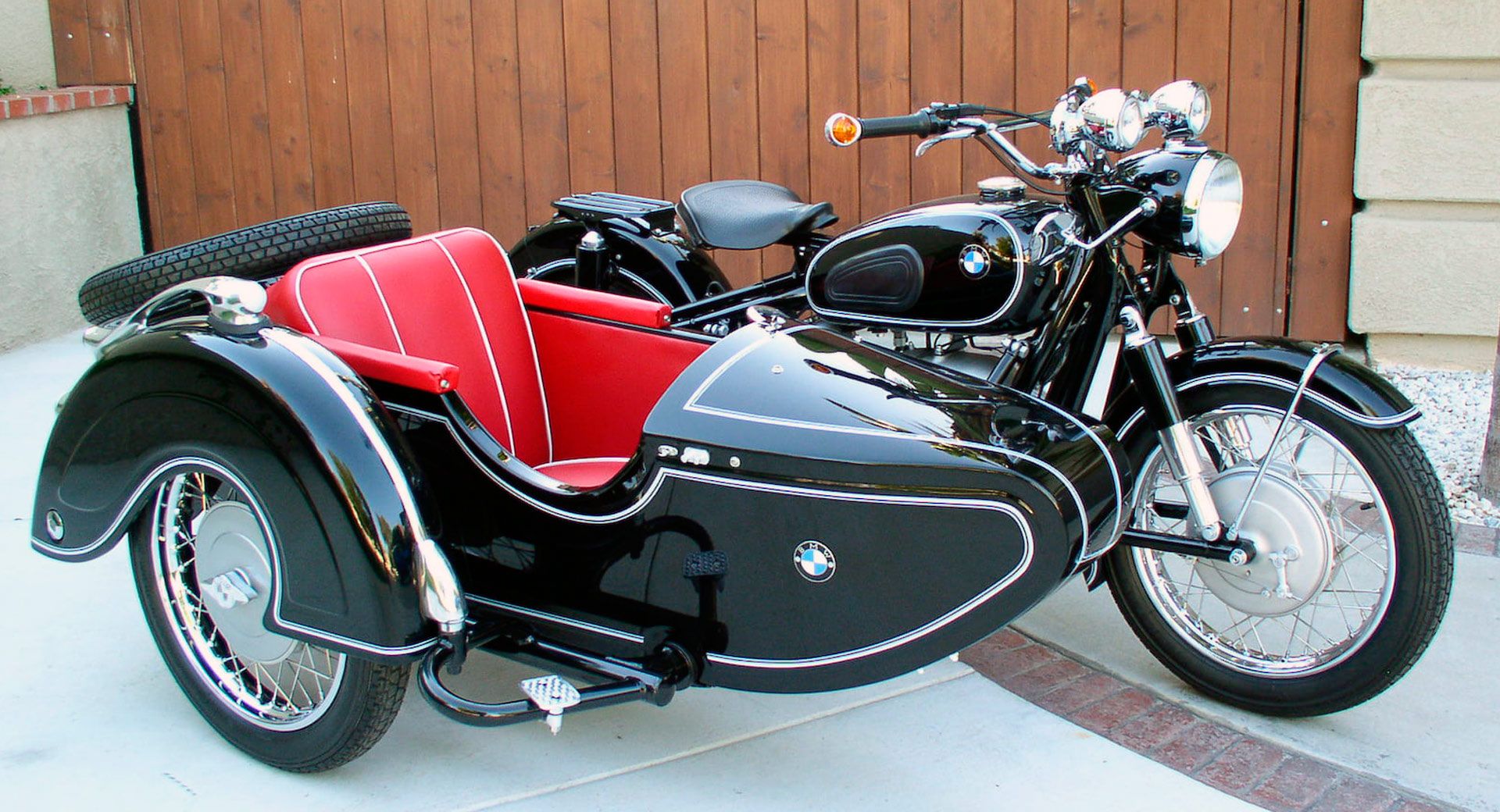In this bright daylight color photograph, a pristine black BMW motorcycle with a sidecar is prominently displayed on a cement sidewalk in front of a brown wooden garage door. The sidewalk features a strip of red bricks running through its center. The motorcycle boasts a sleek design with chrome accents and a leather panhead seat, accompanied by a luggage rack on the back. Its front is equipped with three lights: a large black-encased center light flanked by two smaller lights encased in silver. Both the motorcycle and the sidecar prominently display the iconic blue and white BMW logo. The black sidecar includes a chrome-trimmed step for access, leading into an interior adorned with red leather upholstery and white stripes. A spare tire is mounted on the back of the sidecar. Surrounding the scene is a vertical wooden fence and various wall features including a stone column and a plastered wall with a red brick top, adding depth to the outdoor setting. The entire vehicle ensemble appears immaculate, with gleaming chrome rims and a polished finish, highlighting the meticulous care it has received.